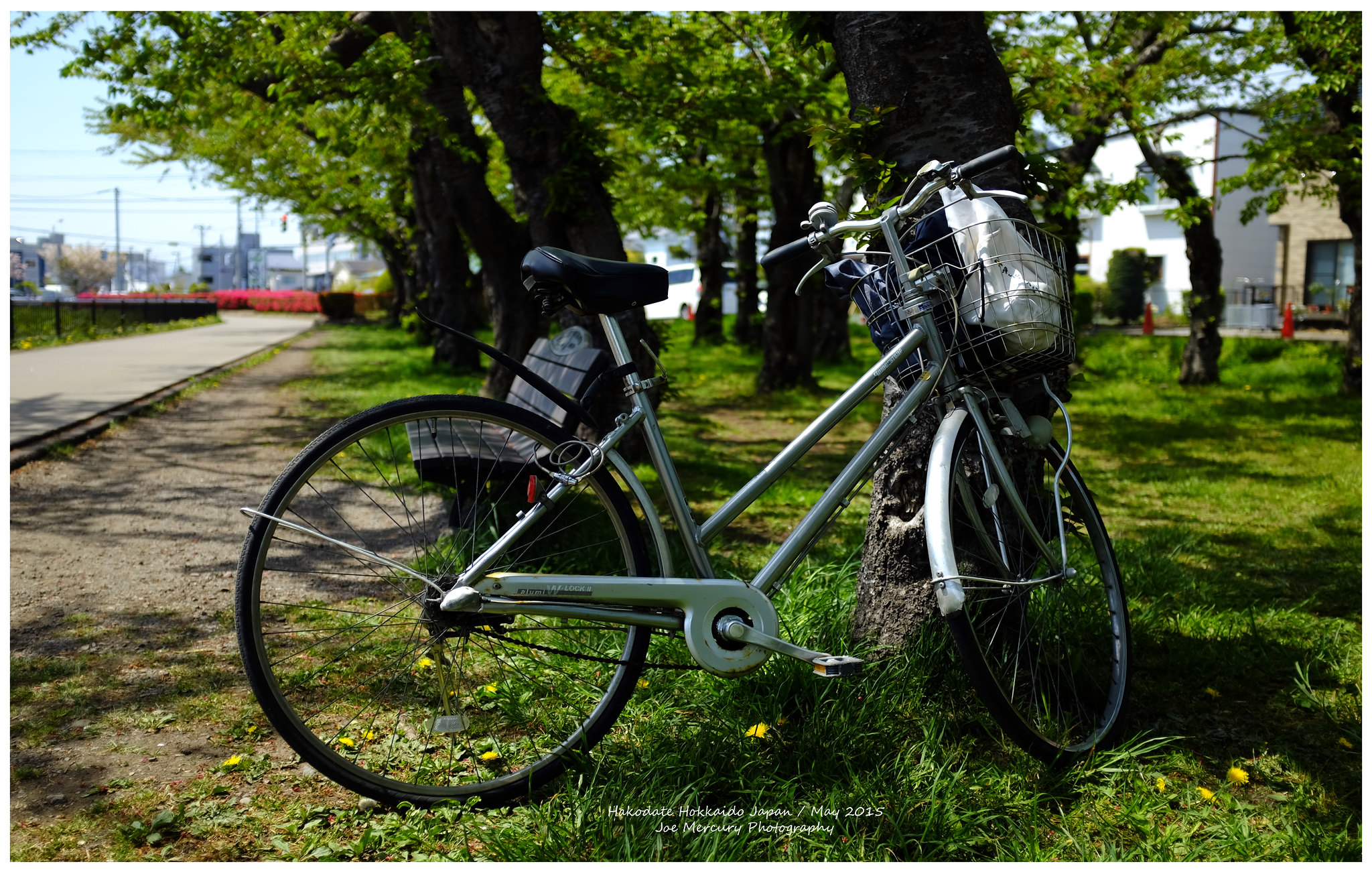In this vibrant outdoor photograph captured by Joe Mercury in May 2015 at Hakodate, Hokkaido, Japan, a woman’s bicycle takes center stage. The bicycle, with its 26-inch tires, features a gray front fender but lacks a back fender. It is equipped with a bell on the handlebar and a metal front basket that holds both a black and a white bag. Positioned against the trunk of a tree with lush green leaves, the bike rests on a patch of grass sprinkled with dandelions, with soil visible behind it.

In the background, there is a white two-story building and a brown brick building, each accompanied by a trash can and a fire hydrant. Further back, the scene extends to a cityscape with additional structures and street elements, including a streetlight, walkway, black fence, and red flowers reminiscent of a park. On the left side of the image, distant buildings and what might be red barrels are seen. A black bench sits behind the bicycle, enhancing the quaint, park-like atmosphere of the scene. The bottom of the image bears the text: "Hakodate Hokkaido, Japan / May 2015 Joe Mercury Photography."